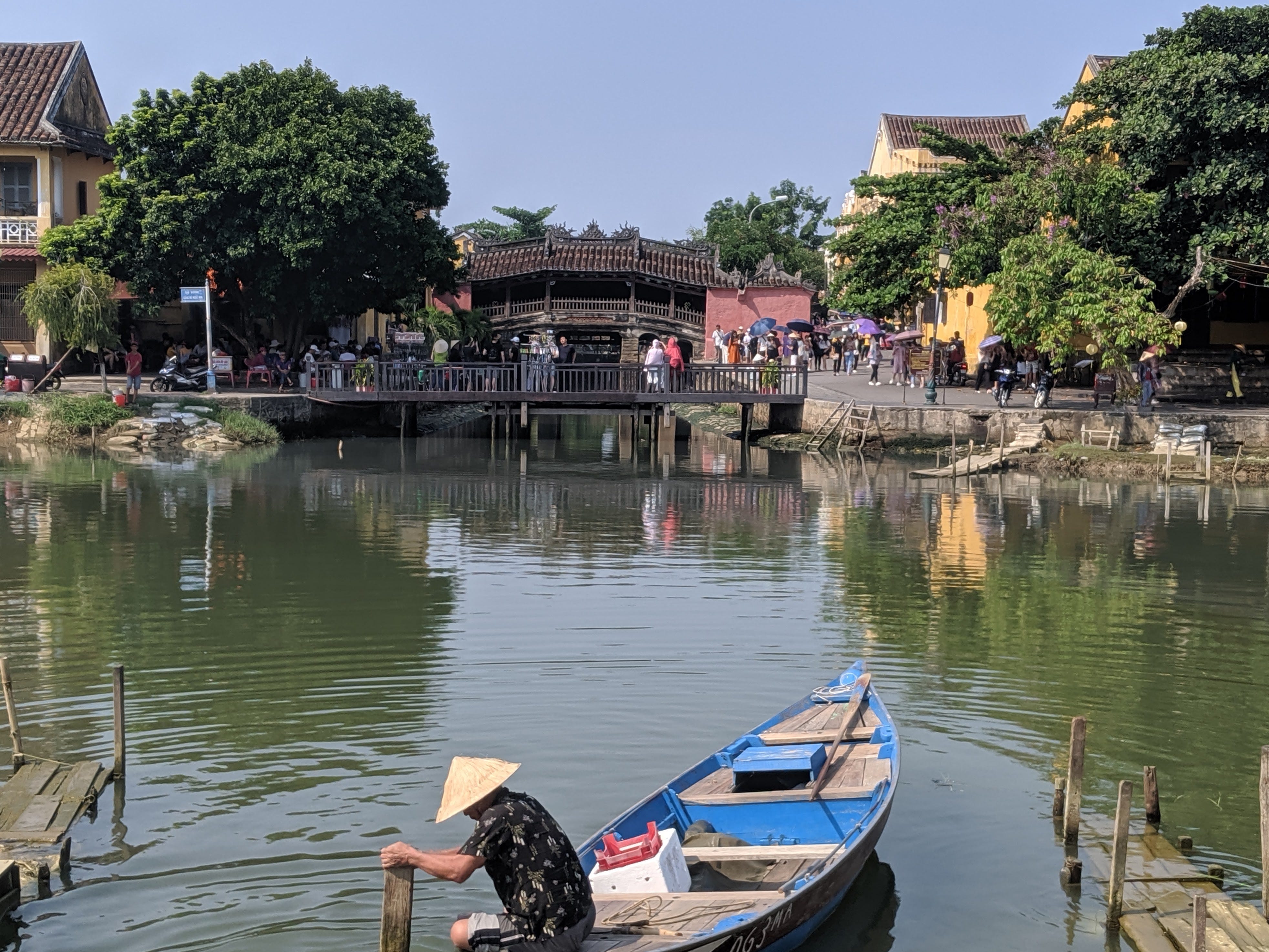This photograph captures a serene waterway, likely in a Chinese or Vietnamese town, featuring a man in an iconic conical hat sitting on the back of a boat. The man, holding onto a wooden beam of a pier, is either pushing off or coming in. The tranquil, green-tinged waterway is framed by lush, verdant trees on both sides, creating a picturesque setting.

In the background, a prominent wooden brown bridge spans the water, permitting numerous people to traverse from one side to the other. Many people stand on the bridge, some using parasols to shield themselves from the sun, suggesting it might be a popular tourist spot. The surrounding architecture features classic Asian-style buildings with pointed roofs, painted in hues of pink and almond.

The scene is lively, with various tourists dressed in vibrant colors like white and red, some pointing and taking in the scenery. Docks line parts of the waterway, and the boat the man rides has a blue interior and tan, yellowish drawers, further adding to the detailed tableau of this charming waterscape.